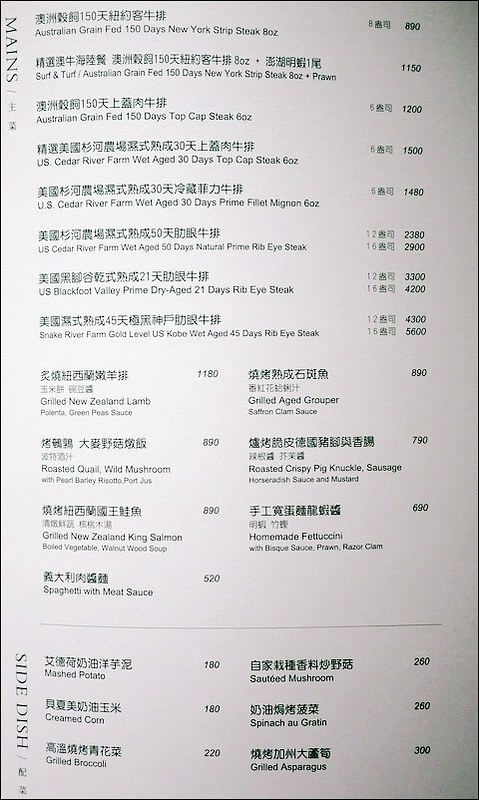The image showcases an Asian menu, meticulously designed with a combination of English and Asian script. The menu is set against a tasteful gray background. Along the left side, the word "Mains" is prominently displayed in English, written vertically. Adjacent to it, there is a section titled "Side Dishes." The Asian script, delicate and intricate, is quite extensive, yet the menu is accommodating to English speakers by providing translations beneath each item.

For instance, the second item listed under the main courses features a detailed description: "Surf and Turf," which includes "Austrian grain-fed, 150-day New York Strip steak, 8 ounces." This thorough translation helps diners understand exactly what they are ordering.

Another highlighted dish is "U.S. Cedar River Farm wet-aged, 30-day prime filet mignon," which even specifies the aging period of the meat, aiding diners in making more informed choices.

The side dish section offers a variety of classic options such as traditional mashed potatoes, creamed corn, grilled broccoli, asparagus, spinach au gratin, and sautéed mushrooms.

Furthermore, the menu is considerate of different appetites and budgets by providing prices for different portion sizes, such as a 12-ounce versus a 16-ounce steak, allowing customers to select according to their preference. This detailed and user-friendly approach demonstrates the menu's commitment to authenticity while ensuring clarity and convenience for all patrons.